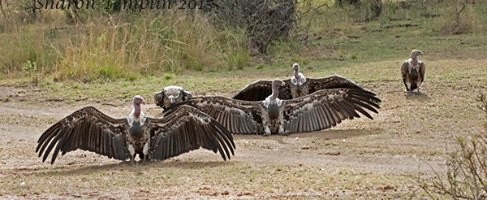This is a small, low-resolution color photograph, taken in landscape format, depicting four large vultures standing on a dried-out creek bed filled with dirt and rocks. The natural background includes some short and tall wild grasses as well as dead shrubs. Three of the vultures are prominently displaying their tremendous wingspans, showcasing their mostly gray feathers and white neck bases, while the fourth vulture, positioned to the right, has its wings folded against its body. There also appears to be a fifth vulture faintly visible on the left. In the upper left-hand corner of the image, partially obscured text reads "Sharon Tempen, 2015." The scene captures the birds in a natural setting, emphasizing their impressive size and the rustic environment they inhabit.